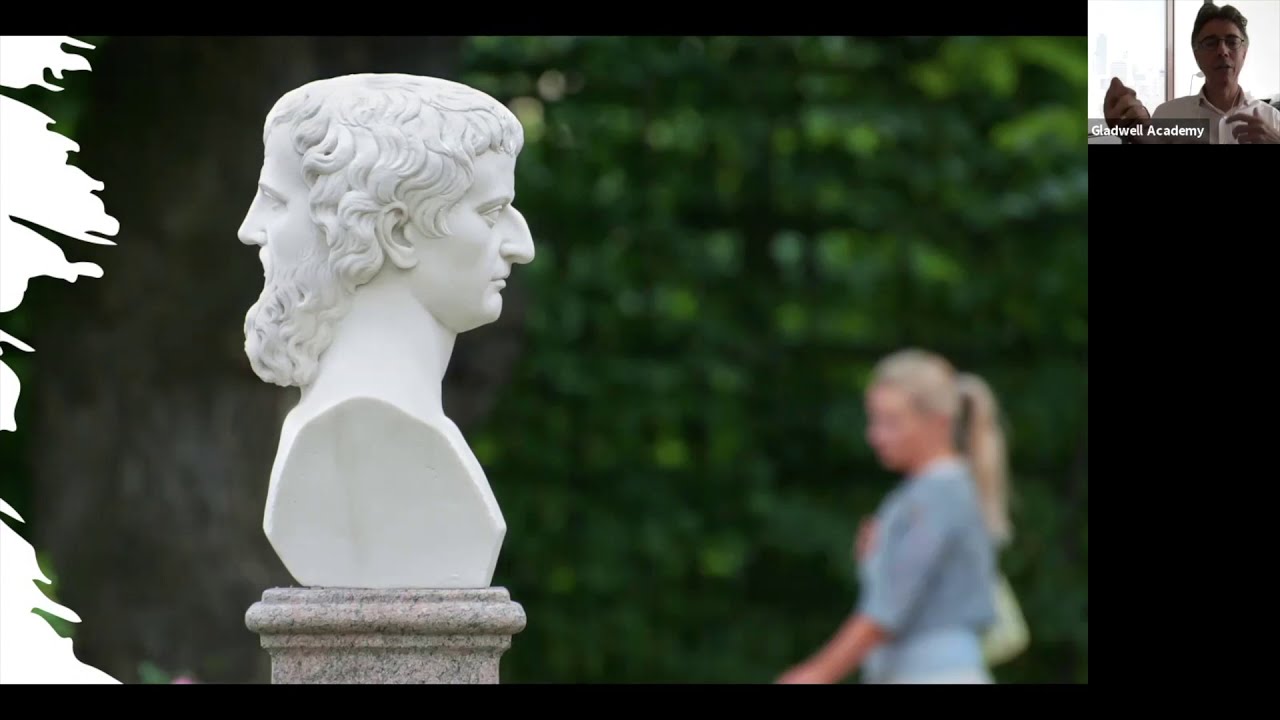The image captures a detailed outdoor scene with a central focus on a dual-faced marble bust resting on a granite pedestal. The statue features two male profiles: the right side depicts a clean-shaven man with an aquiline nose and short hair, while the left shows a bearded man with scraggly hair, their heads joined at the mid-forehead and sharing the same set of hair. In the background, a blonde woman with a ponytail, dressed in a blue sweater, blue top, and possibly a white skirt, walks by with a green purse over her right shoulder. She appears slightly blurred, suggesting motion, and is positioned in front of a green, ivy-covered wall in a park-like setting. Additionally, an inset in the upper right corner features an older man with glasses, wearing a white button-down shirt, mid-discussion on a Zoom call or video stream associated with "Gladwell Academy," evident from the labeling beneath his image.